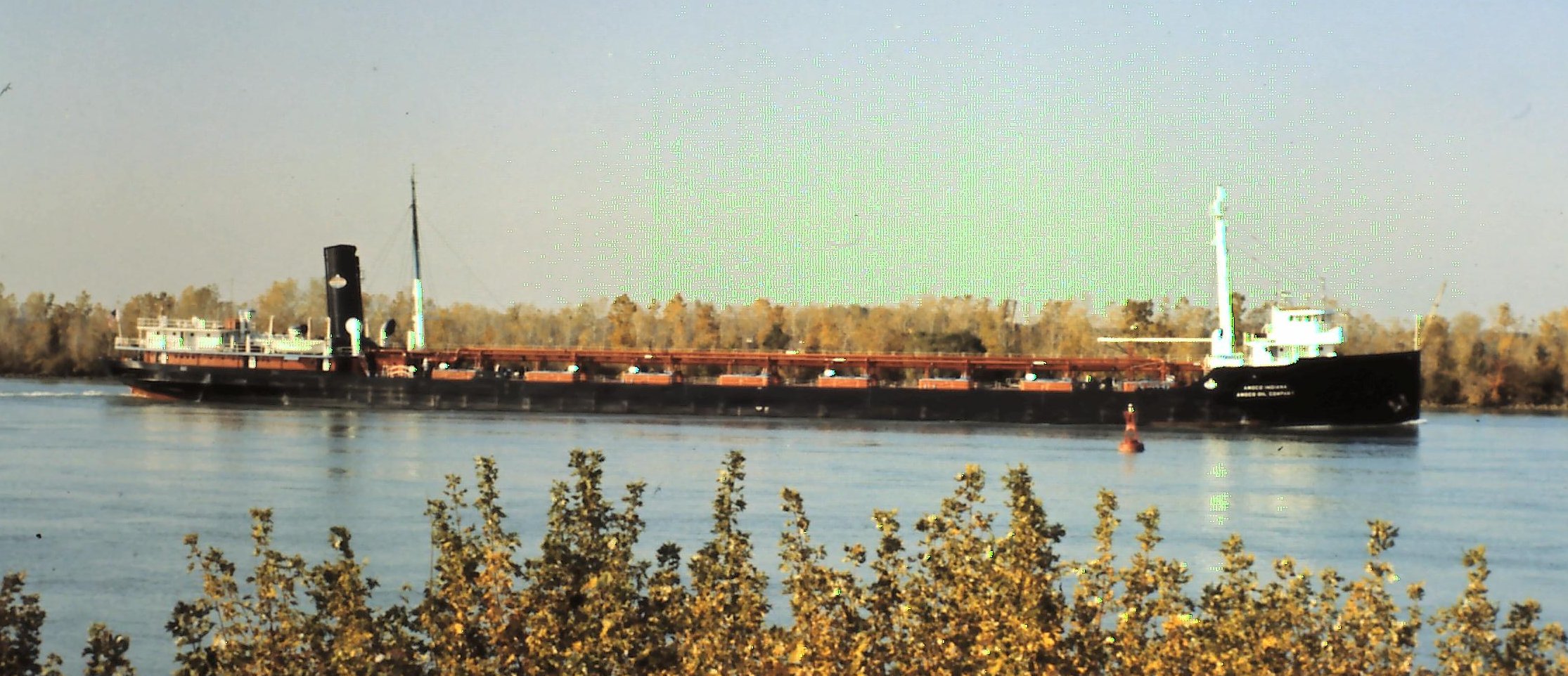A long black steamship glides calmly on a light blue, still body of water, reminiscent of a clear canal or river. The sky above mirrors the tranquil water with its light blue hue, though there is a slight tinge of light green reflected in the middle. The steamship, approximately 80 feet in length, features a white pilot house at the front and a black smokestack towards the rear. Its central section contains numerous chambers, likely used for transporting coal, while the deck and cargo areas are painted in a rusty red color. An orange buoy floats beside the ship, adding a splash of color to the serene scene. In the foreground, a dense shrub with short but abundant leaves extends its branches towards the calm water. The picturesque setting is framed by tall shrubs and trees with green leaves on either side of the river, enhancing the natural beauty of the scene.